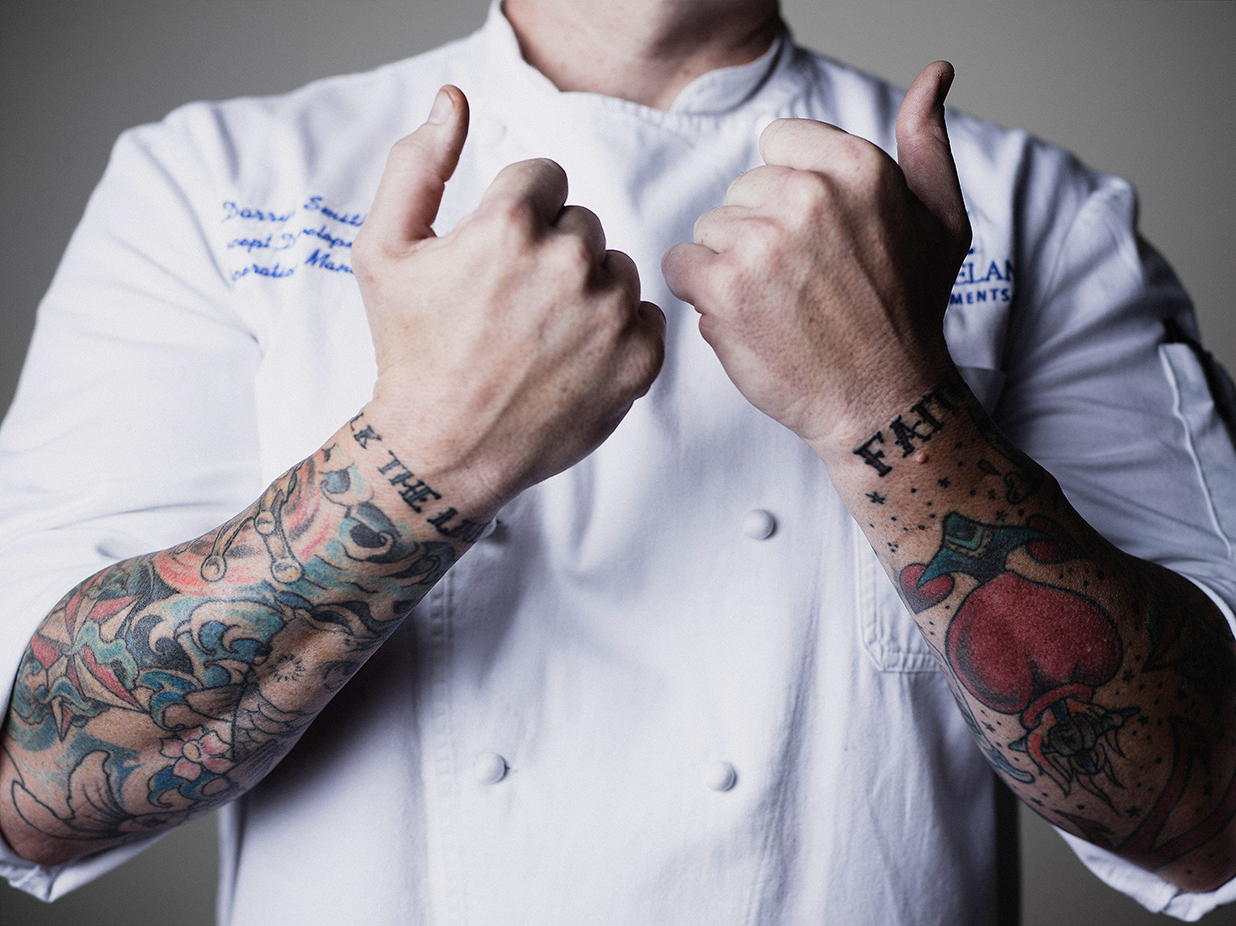This image showcases a man, from the neck down, wearing a white double-breasted chef's uniform. The uniform features three names scripted in blue on the right side, one of which is "Darren," while the other names are unclear. On the left side, there's partially visible blue text reading "E-L-A-N," with the word "M-E-N-T" beneath it. The man is prominently displaying his tattooed arms, raising them in front of his chest with his fists clenched and thumbs out. His left arm showcases a vibrant, swirly design in red and green along with some text near his wrist, where the word "the" is discernible. His right arm is adorned with a traditional heart tattoo, complete with an arrow and flames. Near his right wrist, the word "faith" is visible, although initially obscured and confused with the letters "F-A-T." The tattoos on both arms include elaborate and colorful designs, with his right arm also featuring elements resembling waves and possibly a Japanese-style goldfish or koi fish in blue and black.